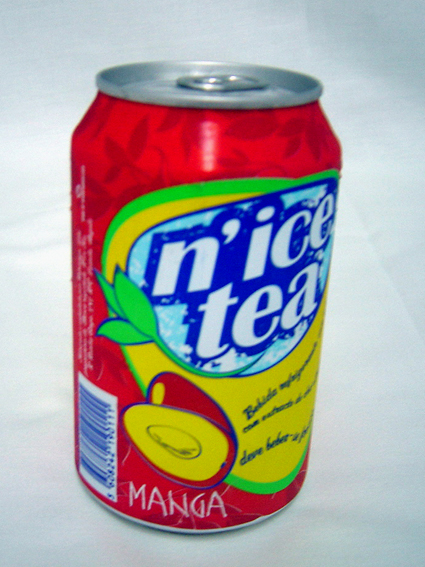The image showcases a vividly detailed soda can labeled "N'Ice Tea." The can's striking red background is adorned with darker red leafy patterns and is prominently centered on what appears to be a pale white marble countertop with a subtle blue tint. The design is accentuated by an abstract, circular-shaped logo that occupies a significant portion of the can, from just below the top all the way to near the bottom. The logo is composed of a lime green ring, a yellow center, and an inner pale blue shape with a darker blue edge. The brand name "Nice Tea" is displayed in large, bold white font within this logo. Below the text, there is a distinctive, stylized image of a mango, hinting at the beverage's flavor. The flavor is further specified with the word "manga" written in clean white letters, positioned just to the right of a barcode at the lower left portion of the can. The entire presentation is complemented by minor details in both English and Spanish, adding to the can's international appeal.